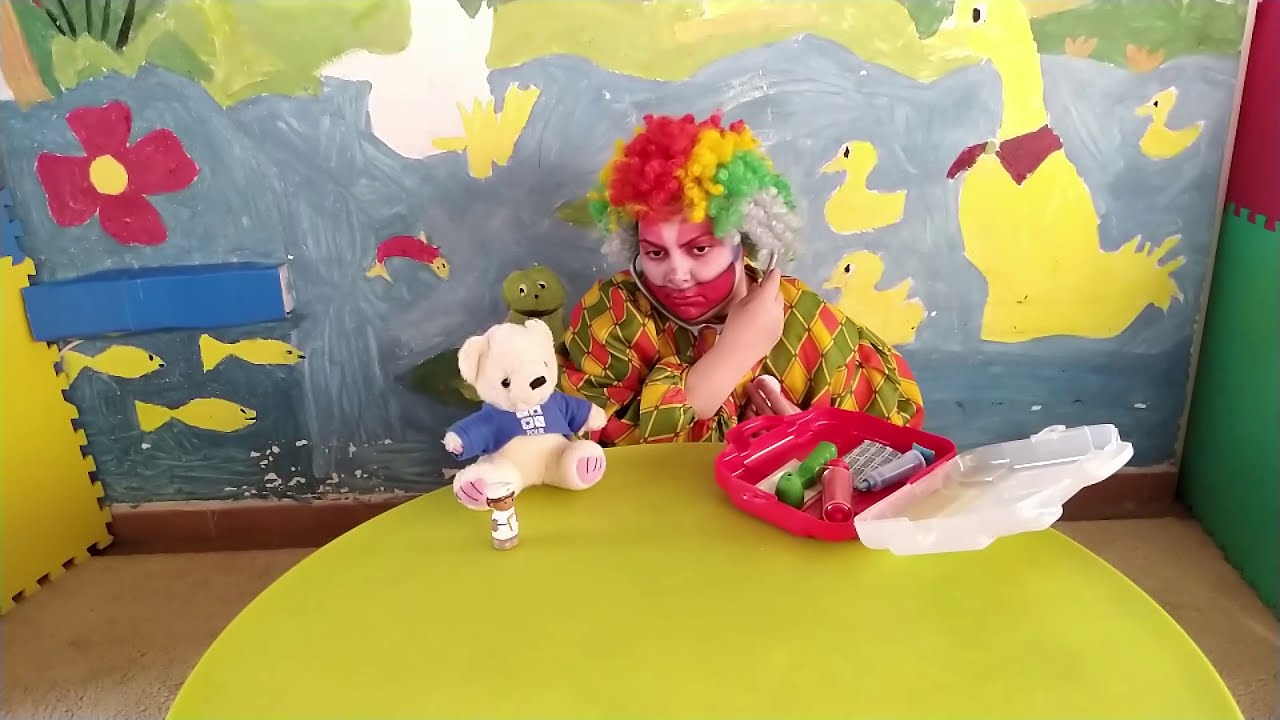The image depicts a photograph taken in a brightly colored children's room, ornately painted with vivid, cartoonish scenes of animals, flowers, and nature, including ducks in a river, colorful fish, and a pink-flowered potted plant. Dominating the lower half of the image is a large, round, yellow table. Seated at the table is a small child dressed as a clown, wearing a multicolored curly wig in red, yellow, green, and white, along with white face paint, a large red mouth, and painted red eyebrows. The child wears a diamond-patterned overshirt in matching vibrant colors. Despite the festive appearance, the child looks sad and conflicted, staring straight ahead. On the table, there's a white teddy bear with a blue shirt and an open plastic container, possibly holding medical supplies, including what might be a smoking piece. Scattered around the bear and container are various unclear accessories. The walls behind the child are painted with lively scenes, creating an overall whimsical yet melancholic ambiance.